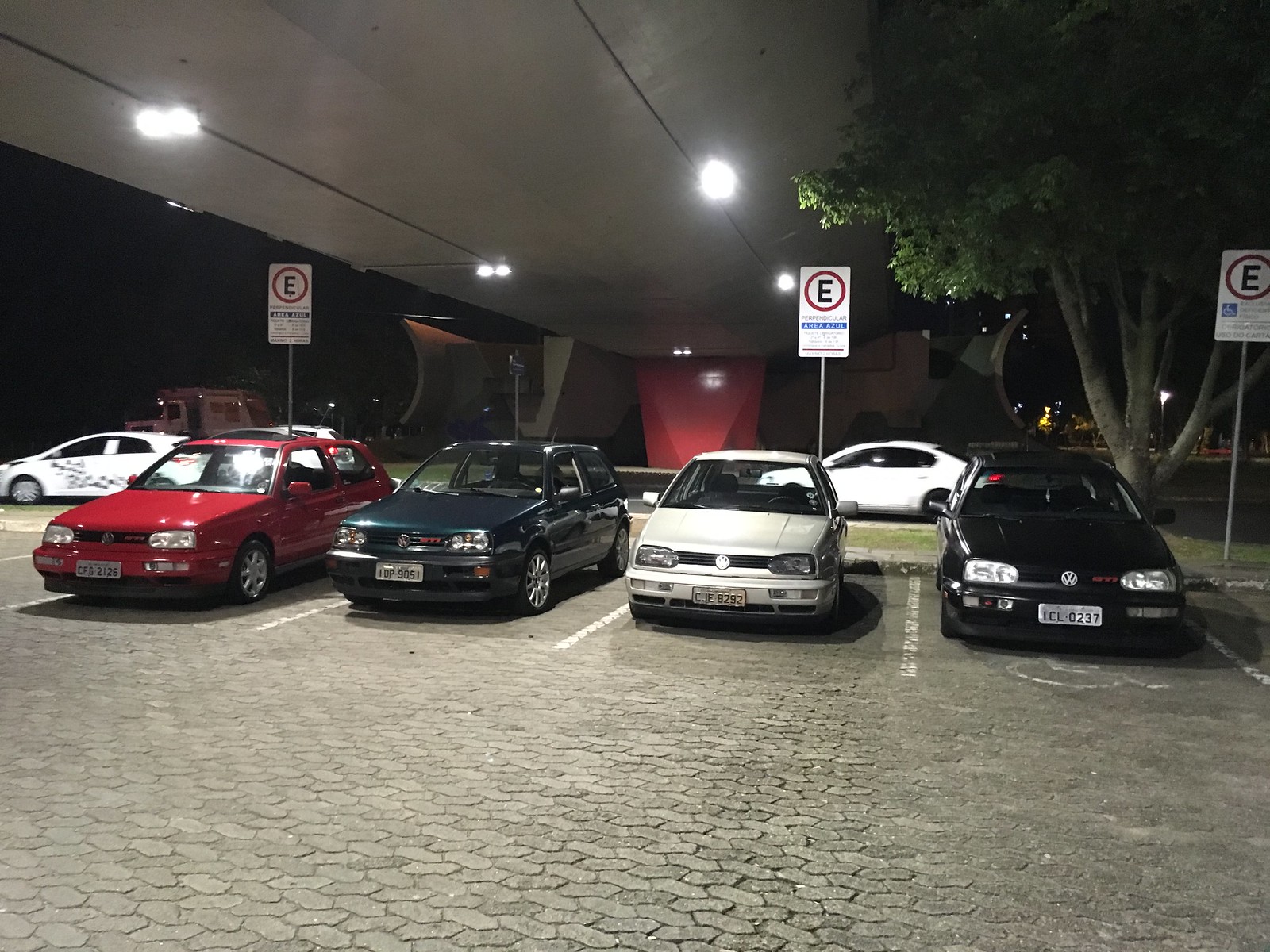This nighttime photograph captures an open parking area beneath a large structure, possibly a highway or the lower level of a building. The dark cobblestone lot holds four primary parked cars: a red car on the far left, followed by a dark blue (or dark green) one, then a white car, and finally a black vehicle. All four are parked with their rear ends to the sidewalk. 

Above each car, there are three identical "No Parking" signs featuring a black 'E' inside a red circle, affixed directly above the black, white, and red cars. To the left of the frame, a white car adorned with side decorations is positioned off to the side of the red car. Across the median, there’s another white car parked perpendicularly on the street curb, appearing to be in motion.

The background shows an exposed outer area; you can see a tree toward the right and glimpses of the sky and distant streetlights. Out to the far left, beyond the sheltering structure, is a visible truck and another car parked outside. The area is illuminated by bright overhead lights and flanked by a red wall on one side of the apparent building structure, giving a sense of an open but covered parking space.